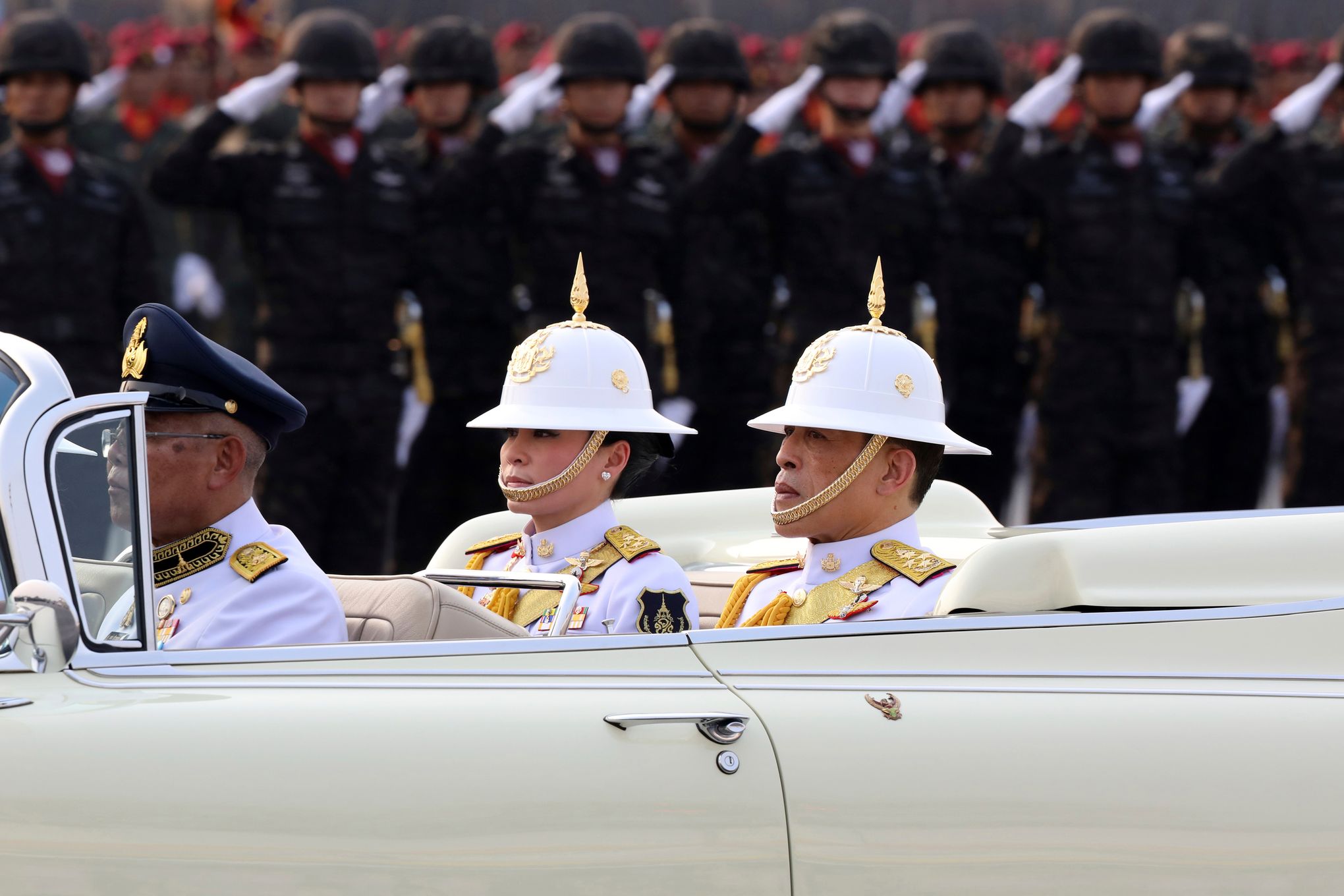In this vibrant outdoor photograph, a cream-colored convertible car is prominently positioned at the bottom side, with three distinguished individuals inside. The driver, seated at the front, wears a light blue military uniform paired with a matching blue commander cap and glasses, looking straight ahead with a sense of duty. In the back seat, two stoic figures don pristine white uniforms adorned with gold badges and insignia, complemented by striking white helmets featuring pointy gold spikes and chin straps. The man on the left back seat wears a black hat with a gold emblem and glasses. Behind the car, a formation of saluting soldiers clad in darker, brown or green military uniforms with black helmets and white gloves can be seen, though their images are blurred, adding depth to the scene. The soldiers salute with their right hands, exuding a sense of respect and formality. The car’s shiny silver handle gleams, hinting at its grandeur. This photograph captures a moment of military precision and honor, highlighting the uniformity and decorum of the occasion.